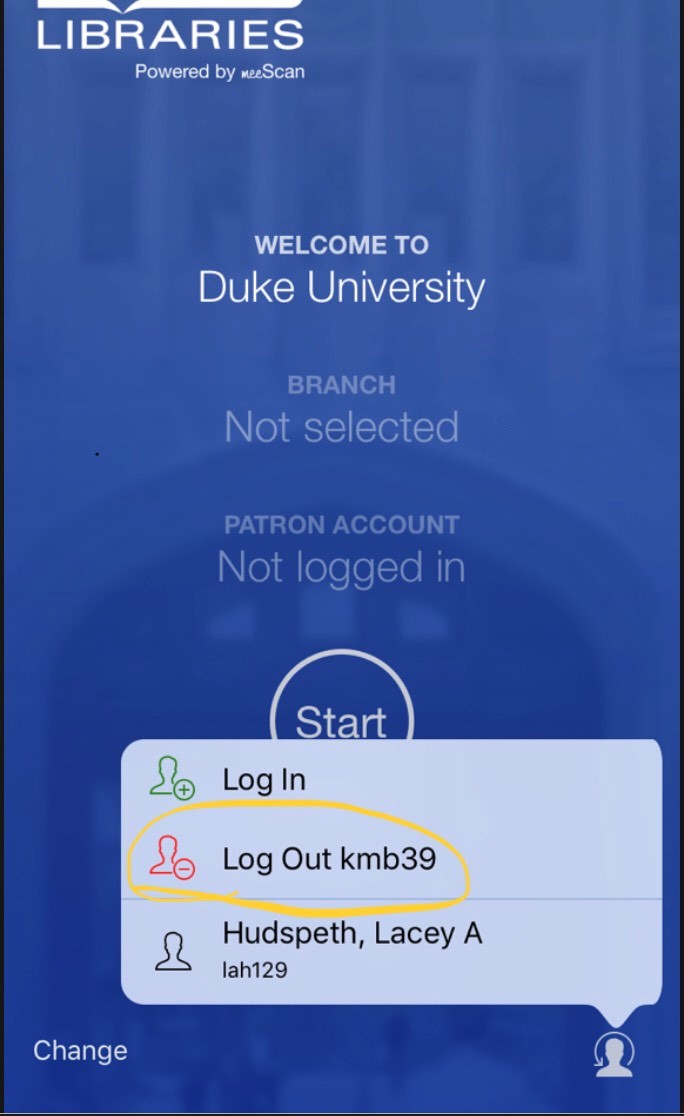The image is a screenshot of a login page featuring a predominantly blue background with white text. In the background, there is a faint, almost transparent image of a grand, white, stately building, showcasing an archway. At the top, the text reads "Libraries powered by MeScan." Below that, it states "Welcome to Duke University" in bold white letters. The site indicates that no branch has been selected and no patron account is logged in. Central to the image, a white circle contains the prompt "Start."

At the bottom portion of the image, there's a pale blue-gray box. Within this box:

- A black text label reads "Login" beside a green icon depicting a person with a plus sign.
- Adjacent to this, another label says "Logout" with a red icon of an abstract person with a minus sign, followed by the identifier "KMB 39," all encircled by a gold ring.
- The final element in the box shows a black icon of a person next to the name "Hudspeth, Lacey A," and the code "L-A-H-1-2-9."

Leading down from this box is a gray silhouette icon of a person with a circle overlay. At the bottom right side of the image, in grayish-white text, it says "Change."